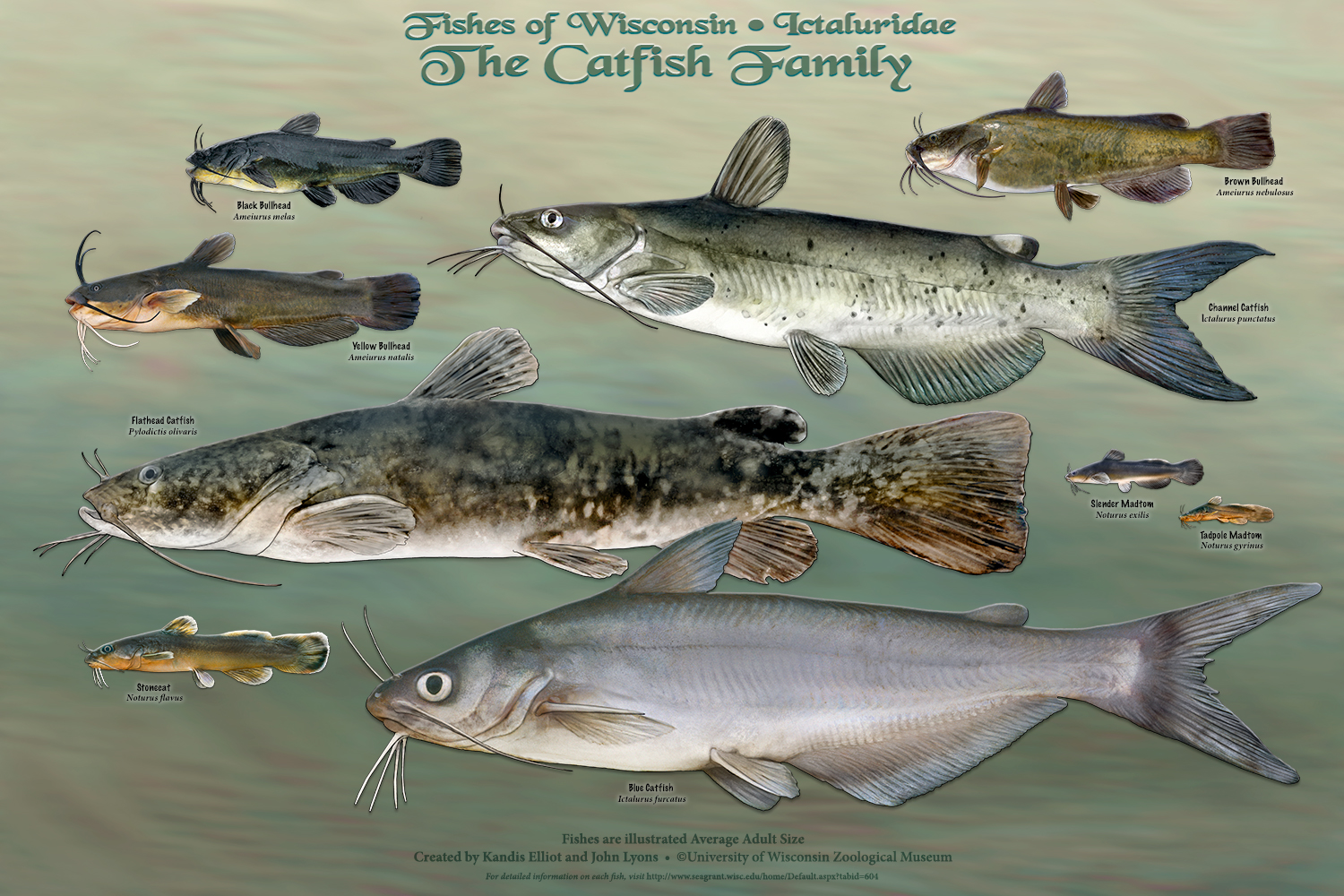The image displays a detailed diagram titled "Fishes of Wisconsin, The Catfish Family," set against a grayish-green background possibly intended to evoke water. The diagram features illustrations of ten distinct varieties of catfish, each oriented towards the left. Though the scientific names and specific descriptions under each fish are in a small, hard-to-read font, the bottom text, which notes that the fishes are illustrated by their average adult sizes, is legible. Prominent in the middle are three large catfish: the bottom one is silver, the middle one is spotted, and the top one is gray with black spots. To the left are three smaller catfishes. On the right, there are two very small catfishes further down and two larger silver catfishes, one of which has black specks. At the top right, another catfish with a greenish-gray body and black specks is present. Different color patterns such as mottling and specific features like white whiskers and blue tails stand out among the catfishes.